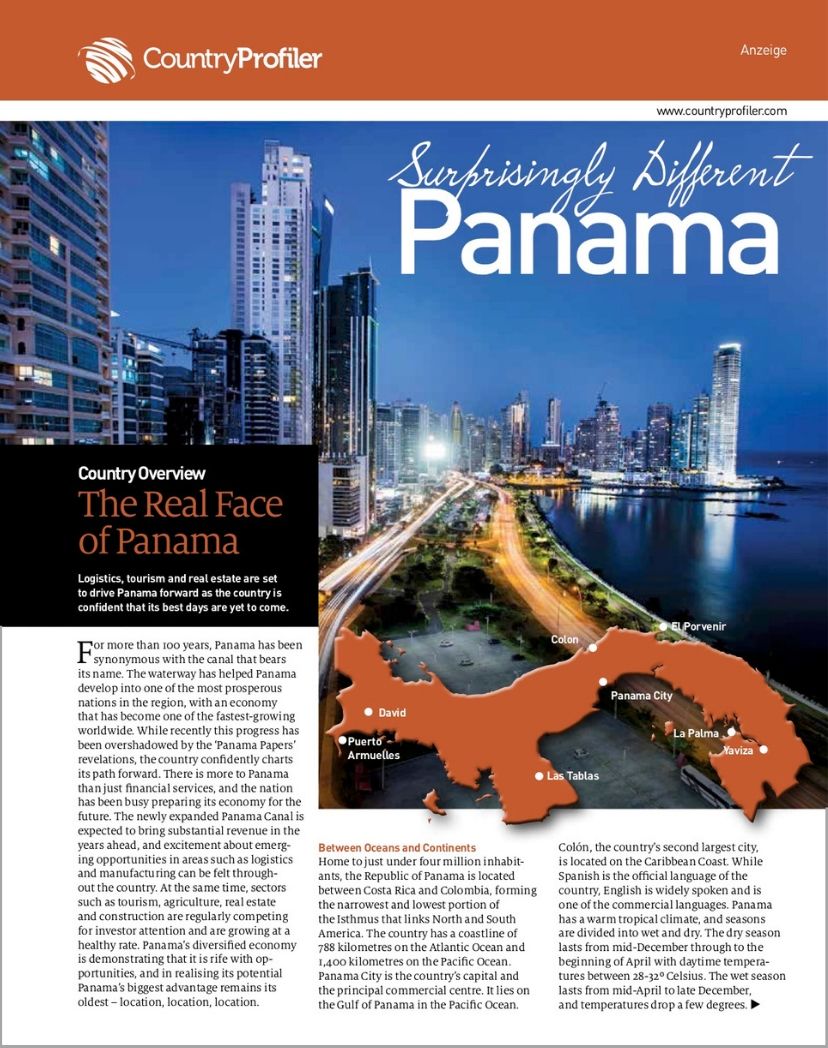In this captivating image, we can see various elements that come together to create a vivid and informative visual. At the very top left, the words "Country Profiler" are prominently displayed next to a logo resembling a white circle encircled by a spear, akin to a planet. The top right corner features text in another language, which appears to be "ANZI", all set against an orange background.

In the top middle section, the phrase "Surprisingly Different Panama" stands out, with "Surprisingly Different" written in cursive and "Panama" in bold white font. This text overlays an actual photograph of what is presumed to be Panama, showcasing a stunning city landscape. On the far right of the image, a large body of water reflects the dazzling city lights. We can also see extensive roads with a distinct orange hue, flanked by lush green areas. The sky above is a stunning, clear blue, contributing to the image's overall vibrancy.

At the bottom right, there is an illustrated map of Panama, colored in orange, pinpointing various locations within the country. In the middle left of the image, we encounter the title of the featured article: "Country Overview: The Real Face of Panama." The article highlights key sectors such as logistics, tourism, and real estate as drivers of Panama's future growth, emphasizing the country's optimism about its forthcoming successes.

This detailed collage effectively captures the essence of Panama, balancing textual information with vivid imagery to provide a comprehensive overview.